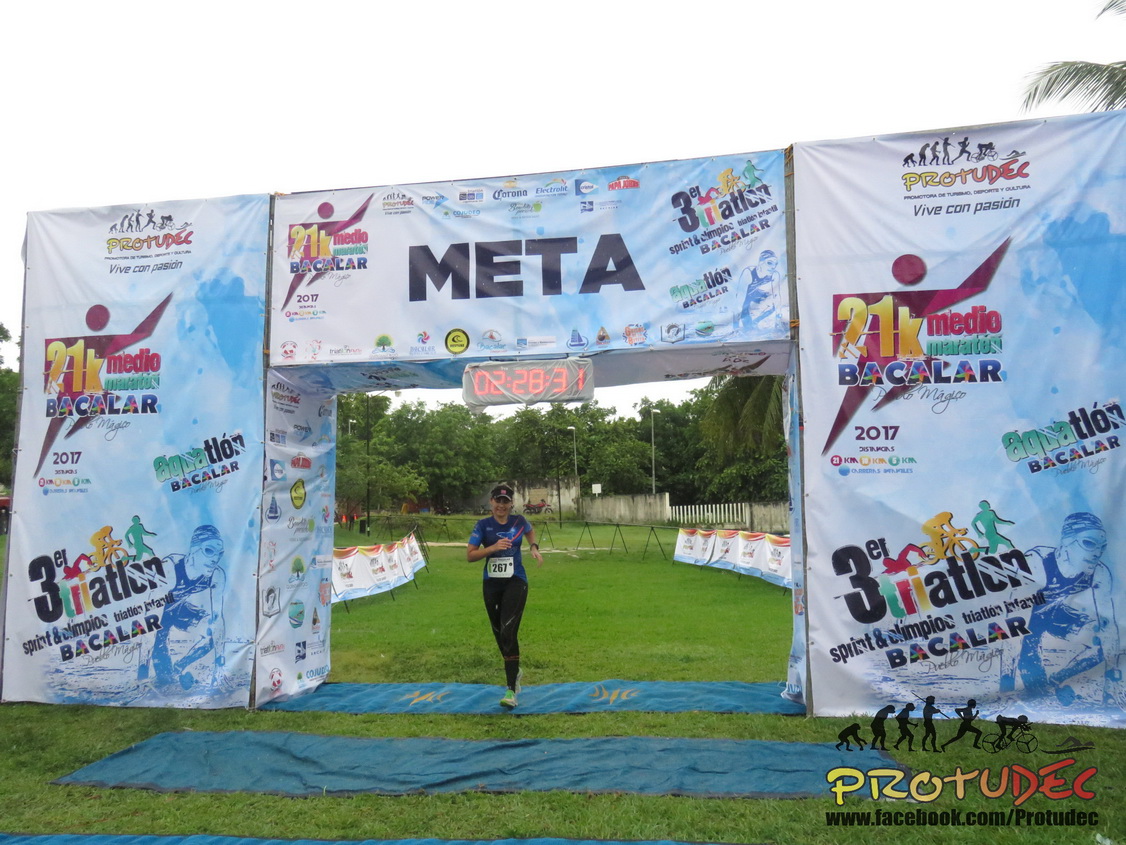In this photograph, a woman runner, donning a blue t-shirt and black pants, races toward the finish line at a triathlon event, smiling with the number 267 pinned to her stomach. She is about to cross a large, light blue gateway structure adorned with various texts and logos, including the prominent word “META” at the center. The timer beneath the archway shows 2 hours, 28 minutes, and 31 seconds. The event takes place on a grass-covered field, with patches of blue cloth scattered across the ground. In the background, fencing adorned with more logos marks the track she just ran. The sky appears white, suggesting either overcast conditions or a bright midday sun. At the bottom right corner of the image, there is a watermarked logo with the words "PROTUDECK" and a Facebook link: www.facebook.com/protrudeck. The scene encapsulates the moment of triumph as the runner nears her goal amidst the supportive and branded atmosphere of the competition.